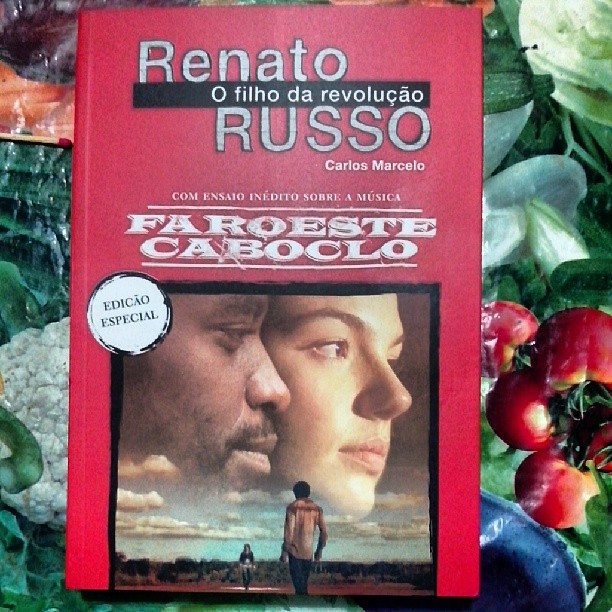The photograph features a red book placed on a table adorned with a tablecloth depicting an assortment of colorful fruits and vegetables, including green, red, and yellow produce such as cauliflower and tomatoes. The book’s cover prominently displays the title "Renato, O Filho da Revolução Russo" by Carlos Marcello, along with texts that read "Com ensaio indédito sobre a música Faroeste Caboclo." There is a circular stamp on the side that reads "Edição Especial." The cover image includes a photograph where two people stand on the ground, while the faces of two more individuals are depicted in the sky above, surrounded by clouds.